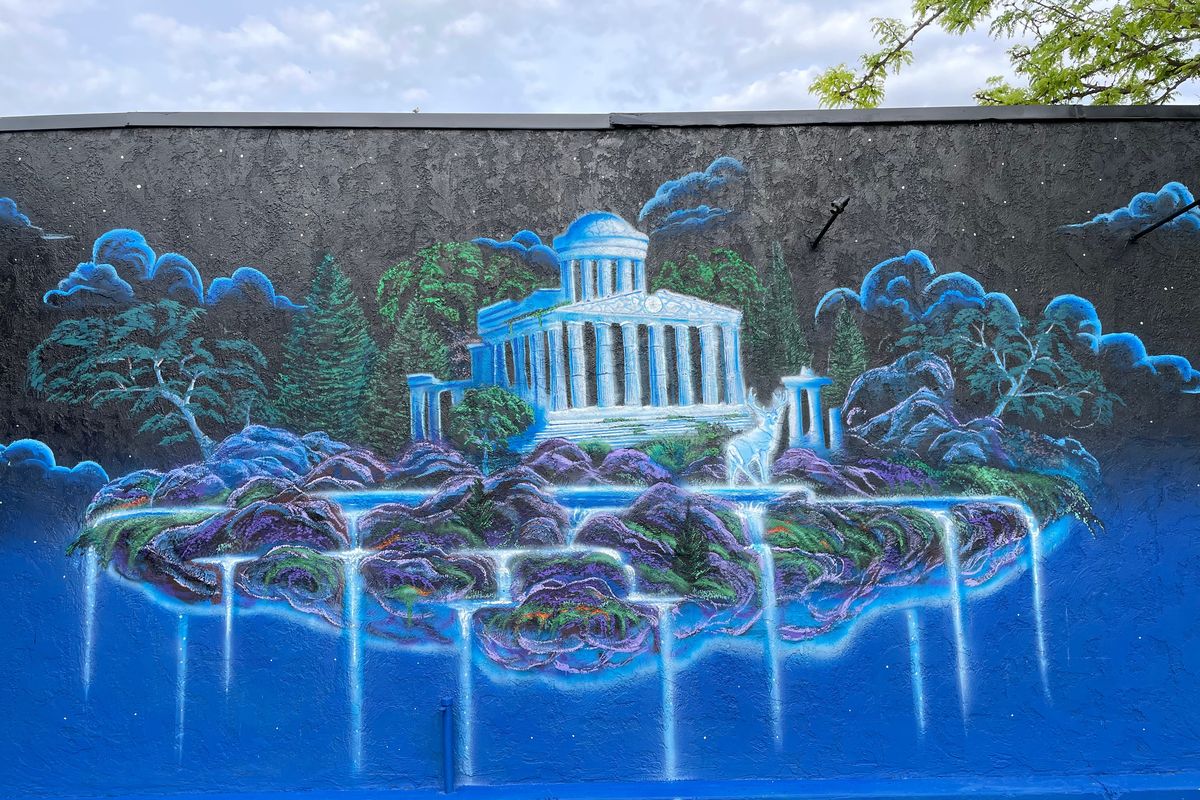This photograph showcases a vividly detailed mural that captures a natural landscape scene with striking clarity. At the bottom, a serene pool of light blue and turquoise water cascades over a rugged rock formation shaded in navy and black, adorned with patches of green moss and lush trees. Above the waterfall, a deeper blue lake is framed by more rocky outcrops in hues of gray and purple. These rocks are interspersed with vibrant green grass, moss, and a mix of darker and lighter green trees, adding a lush, verdant touch to the scene. The mural's backdrop features an ethereal white and pale blue monument standing against a celestial black sky dotted with twinkling white stars. Beyond this, the sky transitions into a soft blue, complementing the vibrant green foliage of a prominent leafy tree. The mural is remarkably vivid and meticulously detailed, making every element easy to discern and appreciate.